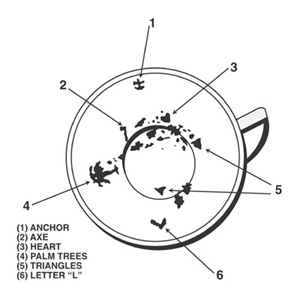The image, drawn in thin black lines on a white background, closely resembles the shape of a mug with a handle, though it is actually a detailed diagram. It features an outer circle and an inner circle, with a handle-like extension on the right side. Inside the circles are six distinct points of interest marked by arrows and numbered consecutively. These numbers correspond to a key located on the lower left side of the diagram. The key details the features of each point: 1 is an anchor, 2 is an axe, 3 is a heart, 4 are palm trees, 5 are triangles, and 6 is a letter 'L' in quotes. These objects are depicted as small, dark gray to black icons within the circles. The entire diagram is encapsulated by a black border, emphasizing its intricate design and focus on the numbered elements within.